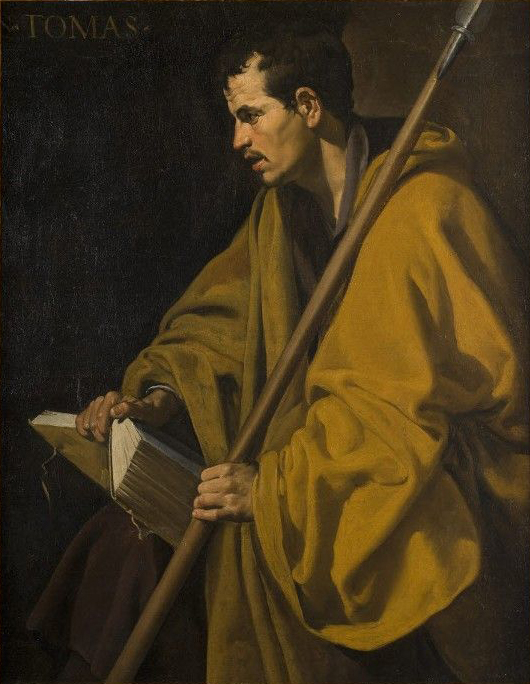In this detailed and expertly rendered painting, we see a man seated and facing sideways, his head tilted slightly to the left. He has short, dark black hair, a black mustache, and pronounced black eyebrows. His complexion is a dark cream color with some redness over his nose, and his ears are shrouded in shadow. There is a distinct shadow under his jaw and part of his neck, enhancing the depth of the painting. The man is attired in a draped, mustard-colored robe that falls in smooth folds highlighted by careful shading. The focused, realistic texture of the robe suggests a masterful hand at work.

In his left hand, he holds a long, wooden staff that extends from the bottom left of the painting to the upper right, resting it on his shoulder. His right hand holds an open book with visible white pages, possibly a thick volume like a Bible, though his gaze is directed elsewhere, suggesting a contemplative or serious demeanor. The background of the painting is dark, providing stark contrast and drawing attention to the figure. In the upper left corner, the name "Thomas" is written in a dark brown hue, further indicating the religious or historic significance of the subject. The painting exudes a timeless quality, with no visible brush strokes, and showcases intricate details and careful rendering, indicative of a skilled Renaissance style.